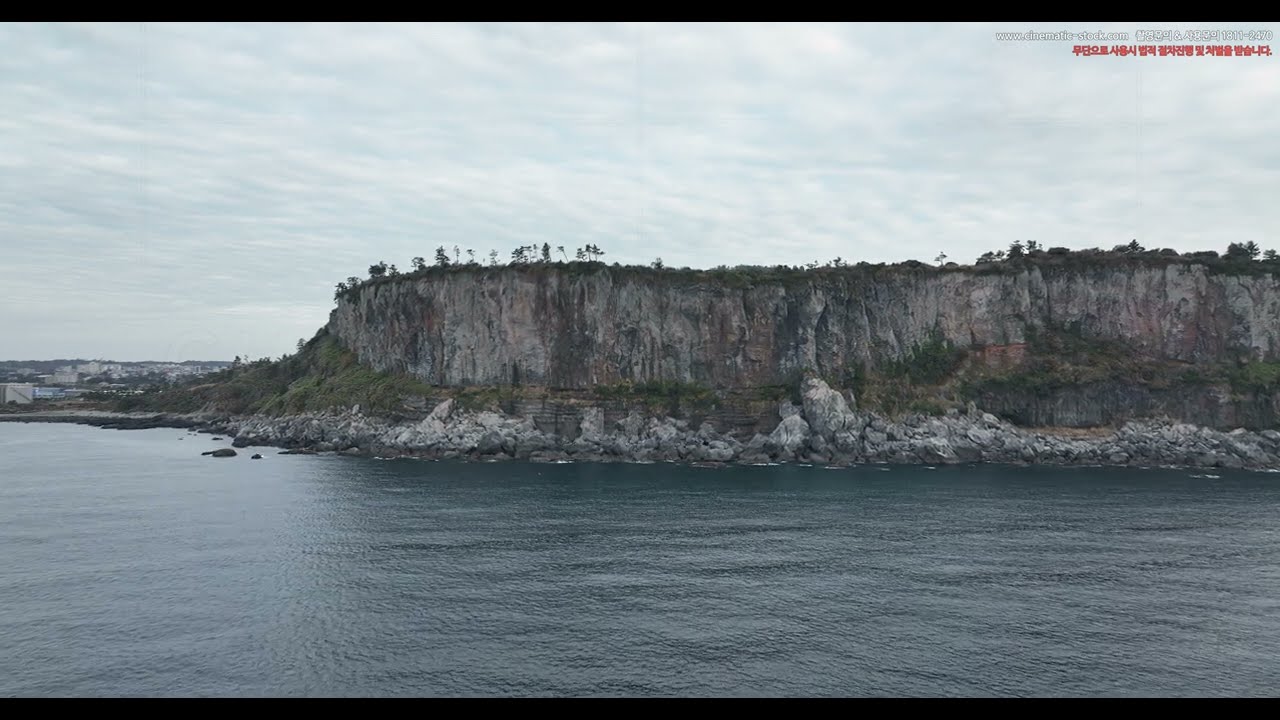The image captures a serene ocean setting dominated by a striking peninsula jutting into the water. The focal point is a large, flat-topped rock formation, partially covered in greenery and foliage, with a few scattered trees crowning its summit. The rocky base descends steeply, making it inaccessible without climbing equipment. To the left in the distance, there's evidence of human habitation, possibly housing developments or a small industrial area, hinting that this formation is part of the mainland rather than a standalone island.

The ocean itself is calm and dark blue, reflecting the overcast sky above. Thick clouds dominate the sky, allowing very little blue to peek through, casting a gray tone over the scene. At the top right of the image, some small white and red text can be seen, though it's too indistinct to read and appears to be in a non-English script. Rocks and stone debris line the shoreline, likely fallen from the cliff due to erosion over time. The entire scene exudes a tranquil yet somewhat desolate atmosphere, beautifully capturing the interplay between natural formations and subtle hints of human presence.